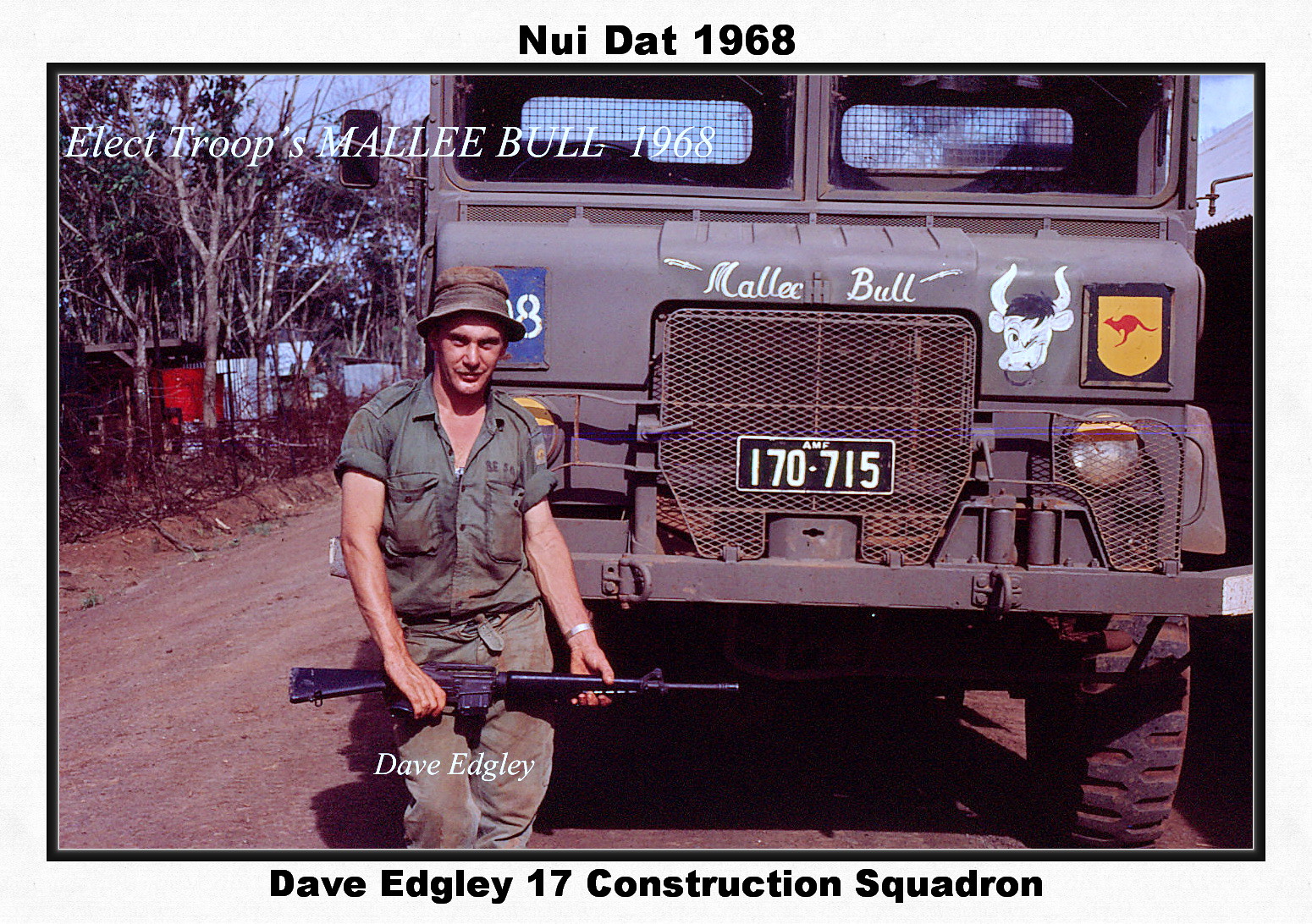This image, likely taken in 1968, features a white male soldier standing in front of a large military truck. He is dressed in a green uniform with sleeves rolled up past his biceps and the neckline open, suggesting warm weather. He wears a brownish-gray bucket hat shading his face, which bears a slight smile. The soldier holds a black assault rifle across his midsection using both hands.

The truck behind him is notable for its large tires and hand-painted decorations. At the top, the truck bears the words "Malik Bull" and "Electroops Malibu 1968." The license plate reads "170715 AMF." Hand-painted on the truck's grill are a cartoonish white bull head with a nose ring and black hair tuft, and a yellow shield featuring a red kangaroo to its right.

The photograph is framed with a thin white border and a thicker black outer border. Text at the top in black font reads "NUI.1968," while the bottom caption identifies the man as "Dave Edgley" from the "17 Construction Squadron." The background hints at a dirt road with trees lining the sides and the sky visible in the upper left corner.